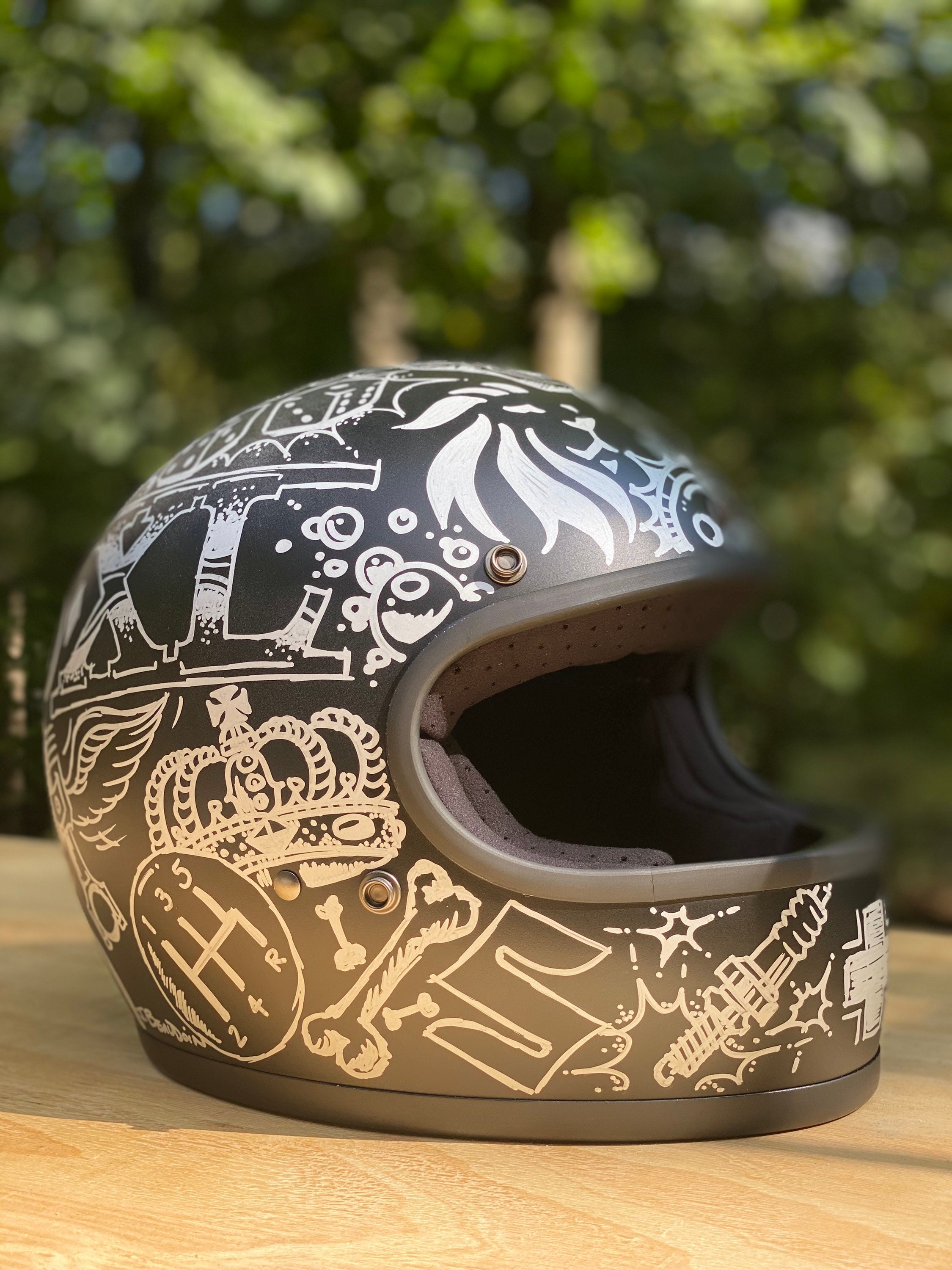This is a detailed up-close photograph of a black motorcycle helmet resting on a light brown wooden table outdoors. The helmet is positioned with its face part facing to the right and takes up most of the image. In the background, there are blurred green trees, indicating a sunny day. The helmet casts a shadow to the left side of the photo. It is adorned with numerous intricate silver designs including a Superman-style "S", dog bones, a detailed royal crown, a winged bird, gears from first through fifth and reverse, flames, a spaceship, a medical cross, bubbles, the letters "XL" wrapping around it, stars, wings, and a spark plug. The predominant colors are the blonde wood, black helmet, silver decorations, and the greenery in the background. The artistic designs on the helmet appear to be done in a marker pen style, creating a visually striking contrast with the black base.